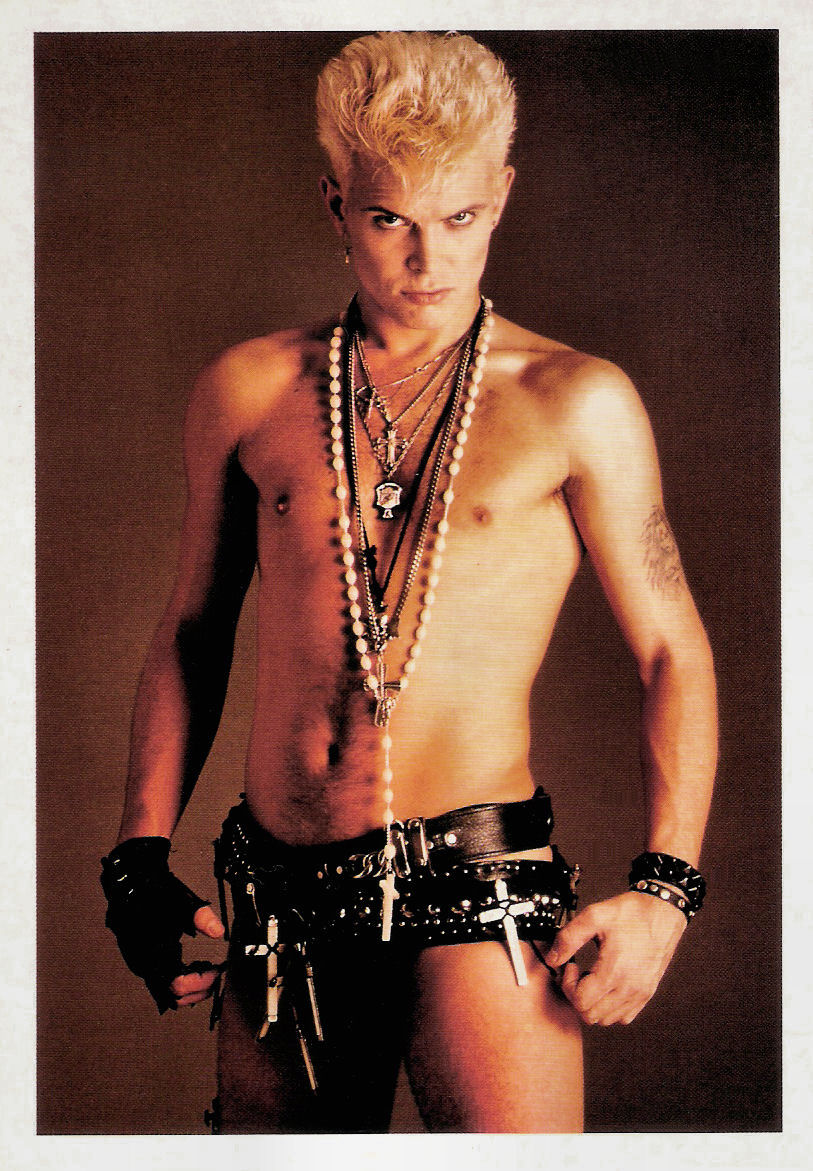This vintage photograph from 1985 features the iconic rock star Billy Idol. He stands at the center of a background in various shades of brown, emanating a bold and charismatic presence. His spiky blonde hair and tanned, muscular physique enhance his seductive look aimed directly at the camera. Billy is almost entirely nude except for black leather underwear, adorned with not one, but two studded leather belts featuring numerous crosses. His right hand sports a fingerless black glove, while his left wrist is decorated with spiked bracelets. A multitude of necklaces, many of which are crucifixes and delicate silver chains, cascade down his chest, some reaching as far as his navel. The absence of text and the simplicity of the brown backdrop emphasize the raw and rebellious energy of the rock star, captured likely in a shoot intended for Rolling Stone magazine.